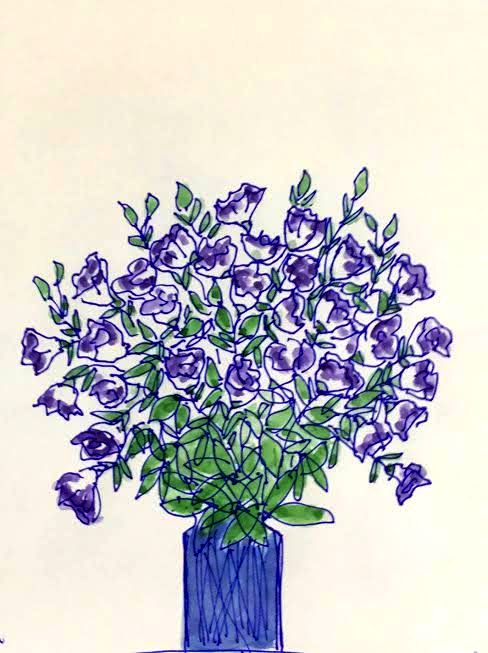This is a color photograph showcasing a child's drawing of a floral arrangement. The artwork is rendered on a pale cream-yellow background. At the bottom of the image, a blue horizontal line is visible, perhaps indicating a surface on which the vase rests. The vase itself is drawn in blue marker, assuming a rectangular shape that narrows slightly towards the top, although the upper portion of the vase is not visible within the frame.

Emerging from the vase is a vibrant bouquet dominated by blue flowers and lush green leaves. The flowers are depicted with a large, almost circular arrangement at the top, with petals tipped in blue and transitioning to a white hue closer to their base. The green leaves appear to spread outward from the mouth of the vase, becoming more dispersed as they extend upwards, giving an impression of being somewhat disjointed from the stems. The stems of the flowers are discernible, providing structure to the overall composition. The drawing is simple yet charming, capturing the innocence and creativity of a young artist.